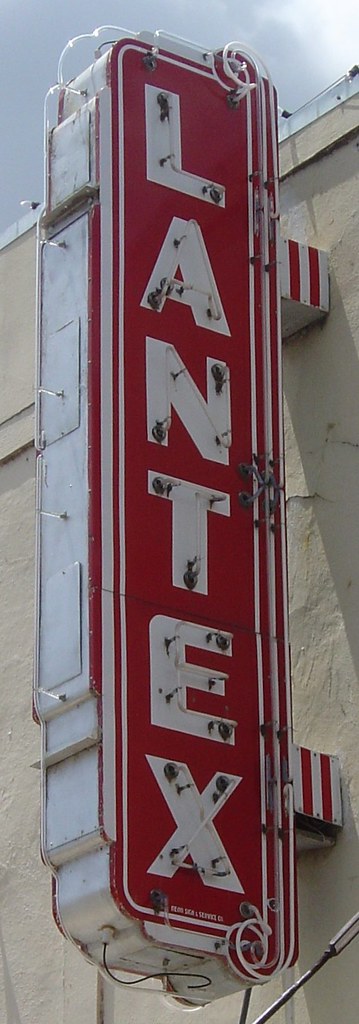This photograph showcases a vintage, vertically oriented sign that dominates the image, which is significantly longer than it is wide. The sign, mounted on the front of a beige building, reads "LANTEX" in white letters against a vivid red background. The distinctive red sign is framed in white, supported by two legs that attach it to the building, adorned with red and white stripes. The frame has an ornate, somewhat retro design reminiscent of the 60s or 70s, and the sign appears to have been illuminated in the past, as evidenced by the holes in the letters and the remnants of wiring. Dark screws punctuate the otherwise white letters, which, along with some dirt and possibly cracked areas, add to the sign's weathered charm. The top portion of the image includes a glimpse of a grey and white cloudy sky, while subtle details such as a small crack and an intentional indent line on the building's facade add texture to the background.